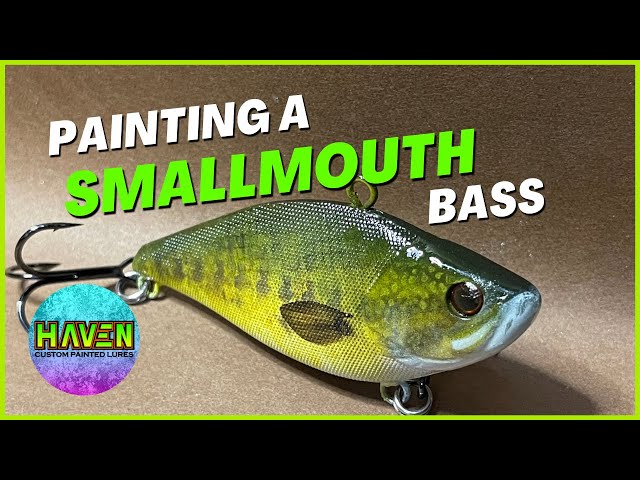This advertisement features an up-close photograph of a meticulously hand-painted fishing lure, designed to resemble a smallmouth bass. The vibrant lure showcases a rich palette of silver and green hues, accentuated by shiny silver highlights, embodying the likeness of a smallmouth bass. Attached to the tail of the lure is a detailed, silver three-pronged fish hook. The advertisement is framed by contrasting black bars at the top and bottom, offering a sleek border to the composition. The background is a textured, heathered brown, giving the ad an earthy, natural feel. Centered above the lure, the words "Painting Ah" are prominently displayed in large white font. The word "Smallmouth" stands out in bold, bright green typography, while "Bass" is rendered in matching white font. In the lower-left corner of the ad, a circular logo featuring blue and purple gradients is visible. The logo contains the word "Haven" in green lettering, with the tagline "Custom Painted Lures" positioned directly below it.